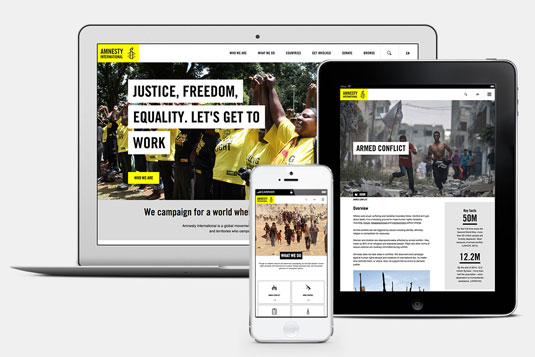The image features a display of three tablets of varying sizes arranged in a layered fashion. The largest tablet at the back is rectangular, partially obscured by a square tablet in front of it, which has a bold black outline. On top of the square tablet is a smaller, vertically oriented tablet. The square tablet is the most visible but contains text that is too small to read clearly.

In the top-left corner of the rectangular tablet, a yellow box prominently displays the word "Amnesty." To its right are some indistinct options. Across the larger rectangular tablet, there are three horizontal bars with bold, black text set against a white background, displaying the phrases: "Justice, Freedom, Equality," followed by "Let's Get to Work." Below these bars, the text reads "We Campaign for World War," accompanied by an image of a diverse group of individuals dressed in yellow and black t-shirts, with their hands raised in a gesture of solidarity and power.

The smallest tablet on top displays a group of people in what appears to be a field or desert environment. To the right of this smaller tablet, the text "Armed Conflict" is visible, showing people running through a city that seems to have been bombed.